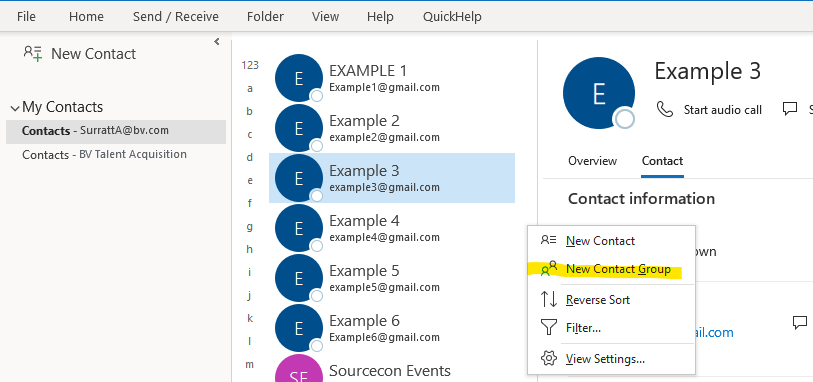The image showcases a user interface with various elements meticulously detailed. At the very top, there is a long gray strip that serves as a menu bar. The menu options are written in a basic Sans Serif font in black, which include: "File," "Home," "Send," "Forward Slash," "Receive," "Folder," "View," "Help," and "QuickHelp," notably lacking a space between "Quick" and "Help."

On the left side of the interface sits a rectangular section with a light gray background. At the top of this section, the heading "New Contact" is displayed in black font. Below this heading, there is an icon depicting a user, followed by two lines and a blue plus sign at the bottom. Beneath this section, "My Contacts" is written in black, with a collapsible arrowhead icon at the bottom left indicating it can be expanded or hidden.

In bold, the word "Contacts" is listed with a space, a dash, and another space preceding it. Following this, in non-bold text, an email format is displayed: "SURRATT A at bv.com." The next line follows a similar format: "Contacts - BV Talent Acquisition."

On the right side of the interface, an extensive list of contacts is visible. The contacts are labeled consecutively as "Example 1," "Example 2," "Example 3," "Example 4," "Example 5," "Example 6," and "SourceCon Events." The third example, "Example 3," is highlighted in light blue, indicating it has been selected.

The right section expands upon the selected contact. It features an icon of a dark blue circle with an "E" in the center. Adjacent to the icon, the name "Example 3" is displayed. At the bottom of this detailed panel, there is a phone icon with the label "Start Audio Call," suggesting an option to initiate an audio call with the selected contact.